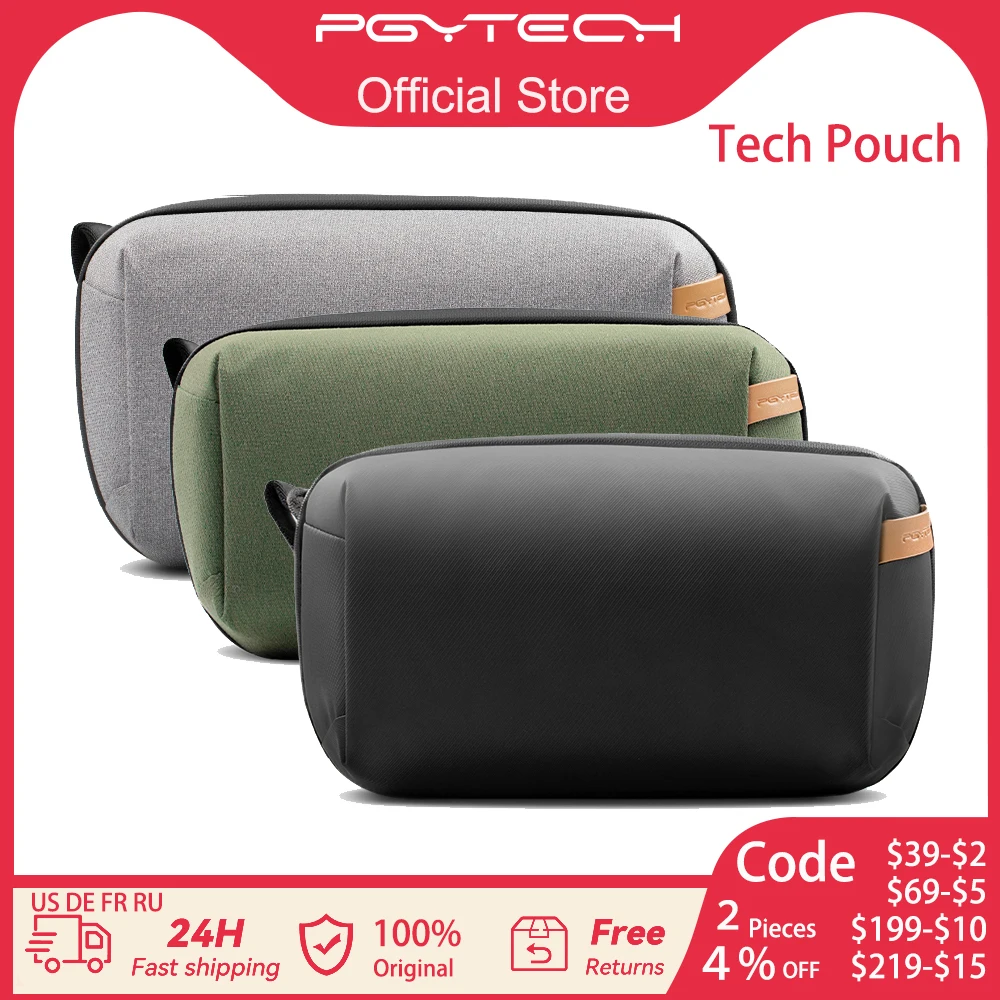The image features a prominently red background with a white rectangular section in the center. At the top of this white section, the text "PGYTECH" is displayed in bold, followed by "Official Store" written underneath in smaller font. To the left (or right, depending on the perspective), the words "Tech Pouch" are written in red. 

The center of the image exhibits three different tech pouches. The one in the back is a light gray color with black trim. The middle pouch is a warm sage green, also with black trim, and features a tan leather loop on the side with another black loop on the back. The front pouch is black, matching the one behind it in design, featuring the same tan leather and black loops.

At the bottom of the image, there is a tan border with the text: "USD-EFRRU, 24 Hour Fast Shipping, 100% Original, Free Returns" prominently displayed. Additionally, on the right side of the image, a red banner states, "Code: 2 Pieces, 4% Off."